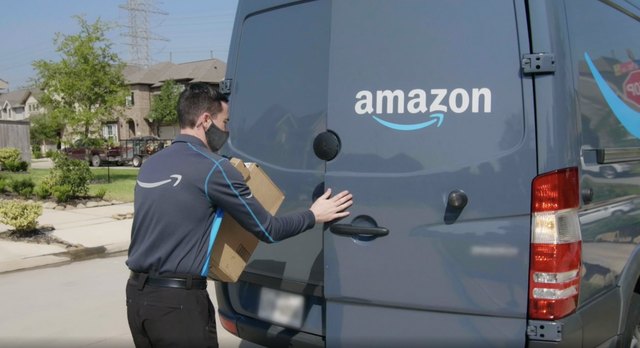In this vibrant suburban scene, an Amazon delivery truck, adorned with the company's unmistakable logo, is parked along a tranquil residential street. A delivery man is captured mid-action, retrieving a package from the back of the van, poised to make a delivery. The color palette brings the image to life with the sleek blue of the truck, the lush green of trees and shrubs, the stoic grey of the pavement, the pristine white houses, and the striking red of the truck's rear lights. Majestic trees and well-maintained bushes frame the background, while several homes add a sense of community to the composition. High power lines traverse the sky above, subtly reminding of modern infrastructure. Bathed in bright, natural light, the scene suggests it is either morning or afternoon, with the sun casting a gentle glow over the suburb, enhancing the sense of everyday serenity and routine.